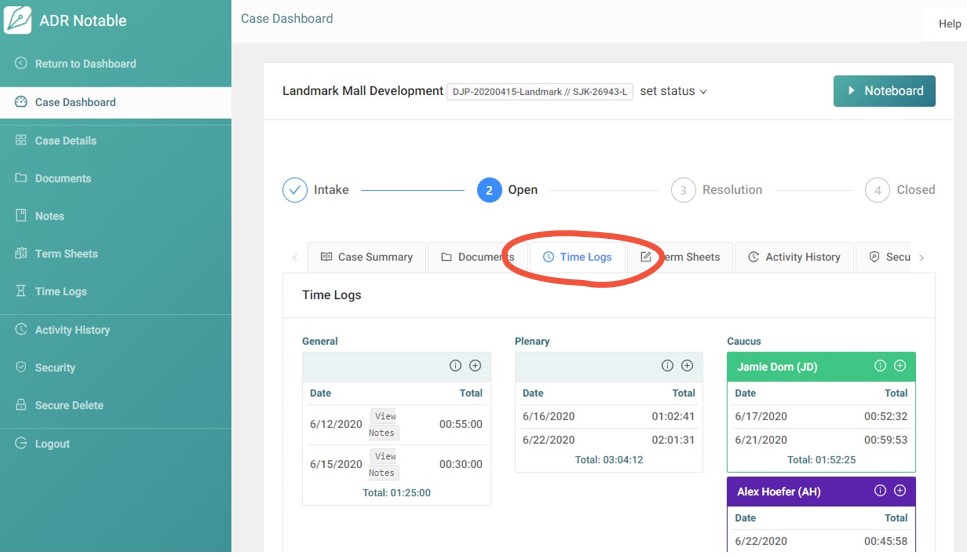This image is a detailed screenshot of the ADR Notable dashboard displayed on a computer screen. The background of the dashboard is primarily white, providing a clean and organized interface. 

On the left side of the screen, a vertical, light blue, almost teal-colored rectangular panel houses the navigation menu. At the top of this panel, there is a white square with a drawn pen nib icon, immediately followed by the words "ADR Notable" in white text. Below this branding, the vertical menu reads in sequence: "Return to Dashboard," "Case Dashboard," "Case Details," "Documents," "Notes," "Term Sheets," "Time Logs," "Activity History," "Security," "Secure Delete," and "Logout."

To the right of this vertical panel, the main section starts with a header titled "Case Dashboard." Directly beneath this header is the project title "Landmark Mall Development," accompanied by a search bar and a drop-down menu labeled "Set Status."

Along the far right of the dashboard, another navigation aid features a directional label that reads "Noteboard" with an arrow pointing to the right, indicating further navigation options. Below this are sequential stages labeled "Intake," "Open," "Resolution," and "Closed."

The central part of the dashboard includes comprehensive information sections: starting with "Case Summary," followed by "Documents," "Time Logs" (highlighted by a red circle for emphasis), "Term Sheets," and "Activity History." 

At the bottom of the screen, there are tabs categorized as "General," "Plenary," and "Caucus," rounding off the interface options available for detailed case management and navigation on the ADR Notable platform.